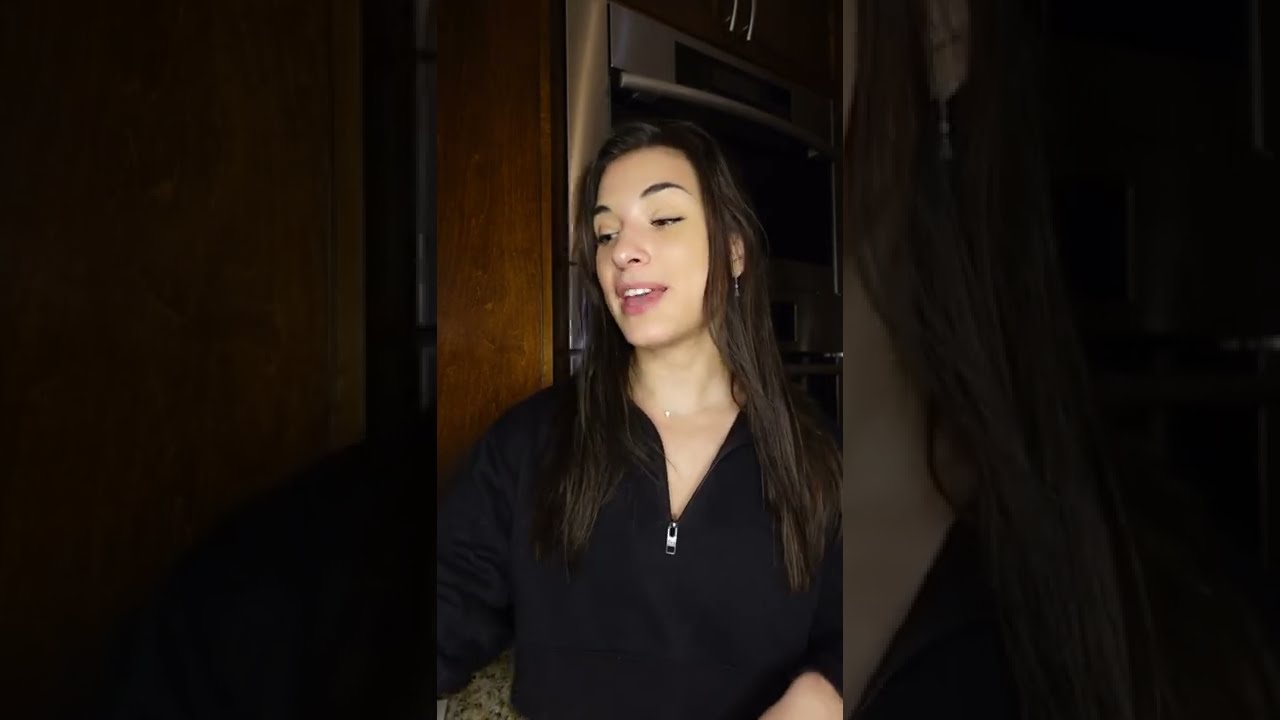In the image, which appears to be a screen grab from a video, a young woman in her 20s is featured. She is wearing a black long-sleeved sweatshirt with a zippered collar that is partially unzipped. Her long dark hair drapes over her shoulders, and she has a small gold necklace around her neck. The woman, with a medium white complexion, appears to be engaged in singing or lip-syncing, as her mouth is open and she is looking slightly towards her right, possibly at the seven o'clock position.

The image composition is divided into three panels, with the center panel being vertically rectangular and flanked by zoomed-in versions of the same image on either side. The overall lighting is dim, with a light source shining on the subject, highlighting her expressive demeanor. She is indoors, and the background features a combination of dark brown wooden structures, possibly a door or paneling, and shelves. There is also a hint of stainless steel appliances and perhaps a monitor, contributing to a cluttered but homely setting.